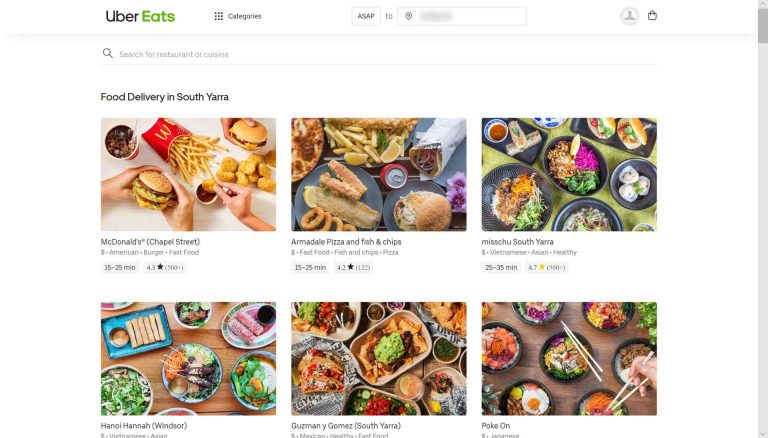This is a detailed screenshot of the Uber Eats website page. 

- **Top Section:**
  - At the top, there's a horizontal white bar spanning across the screen.
  - On the top left, the Uber Eats logo is prominently displayed; "Uber" is in black text, and "Eats" is in green text.
  - To the right of the logo, there is a "Categories" button.

- **Middle Section:**
  - Centrally located are two fields:
    - The first field reads "ASAP".
    - Between the two fields is the numeral "2".
    - The second field has a pin icon and is censored out for privacy reasons.
  - To the right of these fields, there are icons for the user profile and a basket.

- **Below the Top Section:**
  - A light gray section houses a search bar at the top, prompting users to "search for a nearby restaurant or cuisine."

- **Main Content Area:**
  - Below the search bar, the phrase "Food delivery in South Florida" is displayed.
  - Further down, six images of diverse food items are spread out on a table, representing different restaurants:
    - The first three images showcase food from McDonald's, Armadillo Pizza, and Miss Chew.
    - The last three images are associated with a restaurant named Hanoi Hanna.

Each element of the page is clearly organized to guide users smoothly through finding and ordering food online.